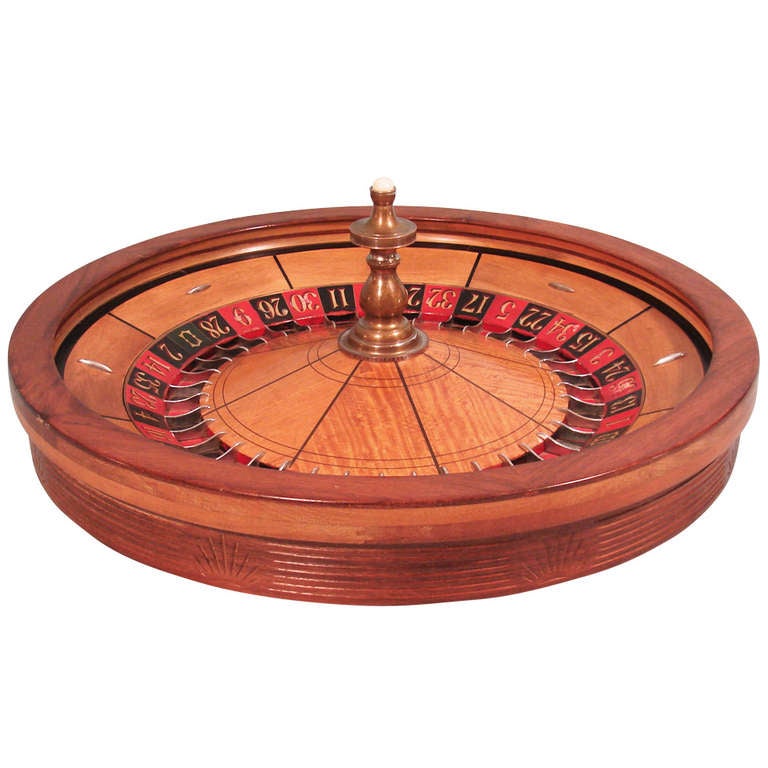The image showcases a meticulously crafted wooden roulette wheel set against a stark white background. The wheel, constructed from two-toned wood, features a darker, flatter top surface and lighter wood accents along the sides and inner sections near the spinning knob. The wood exhibits a polished, well-maintained finish, suggesting either a piece for sale or an artifact from a different era. Encircling the wheel are alternating red and black numbered sections, each finely painted and sectioned off with intricate notches that may serve decorative purposes. The center of the wheel contains a bronze or brass spinner knob, which is the focal point for spinning. Engravings and black painted lines adorn the sides, further enhancing its detailed craftsmanship. The absence of a spinning ball or die preserves the pristine presentation, emphasizing the wheel's professional and polished appearance.